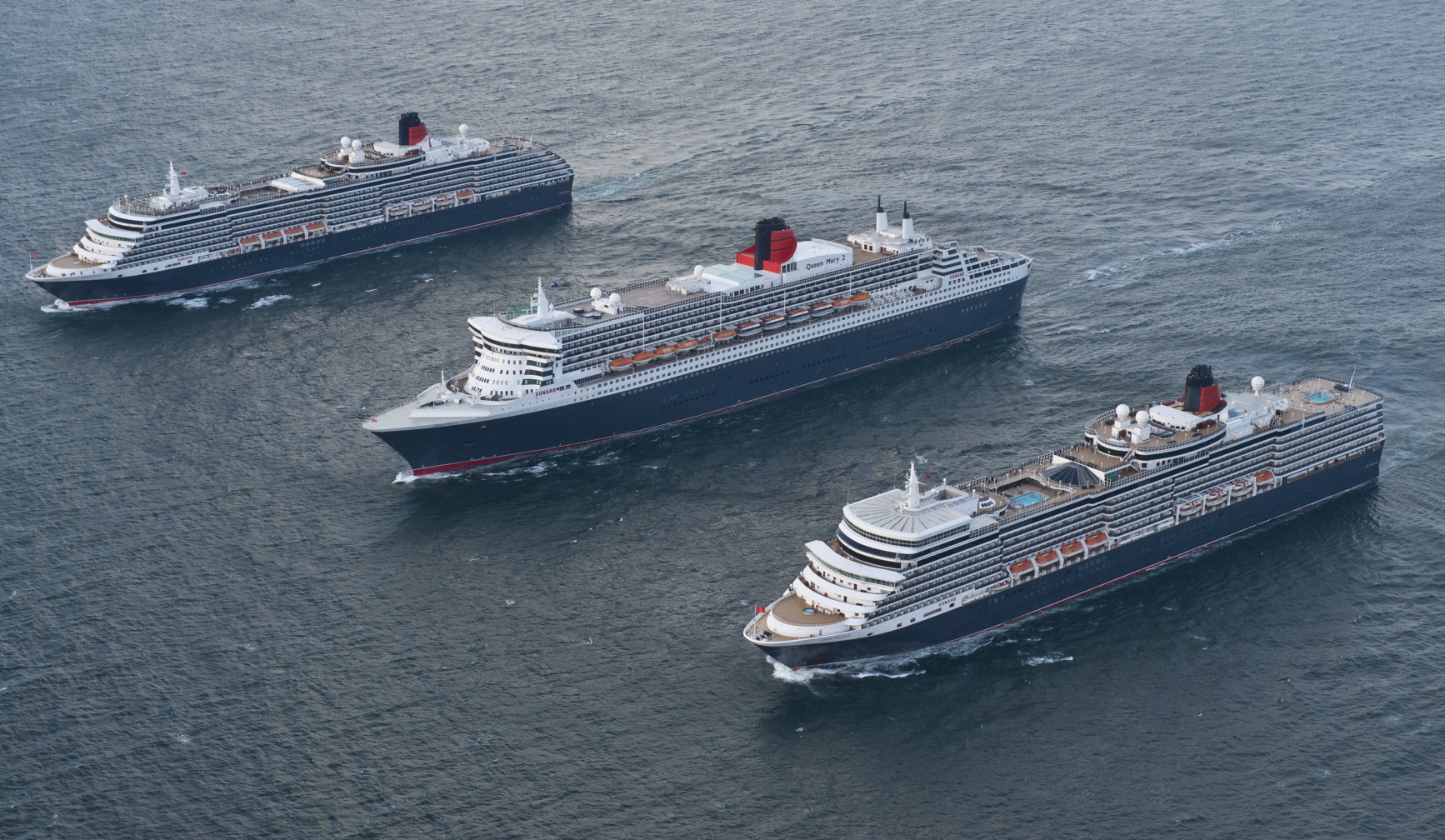This photograph captures a trio of impressive commercial cruise liners navigating the calm, textured blue ocean. The ships, arranged diagonally from the top left to the bottom right, are all facing left and aligned with even spacing. Bathed in bright sunlight, the image has a slight grain and a cyan tint that adds to the scenic, tranquil ambiance of the open sea. Each ship is predominantly white with accents of red and dark blue, featuring a distinctive red and black smokestack at the top, suggesting they belong to the same cruise line.

The most prominent vessel is the middle ship, identifiable by the text "Queen Mary Two" on its upper deck. This ship appears to house more passengers, as indicated by the greater number of orange and white lifeboats. It also seems to be the largest of the three liners. The ship on the bottom right has a visible swimming pool, a light blue square located near the middle, with a second pool possibly situated towards the back. The ships on the top left and the middle do not have visible pools, intensifying the unique charm of the bottom right liner.

All three ships showcase multiple decks and an elegant blend of dark blue at the bottom, red detailing, and a white superstructure, highlighting their grandeur and sophistication against the serene waters.